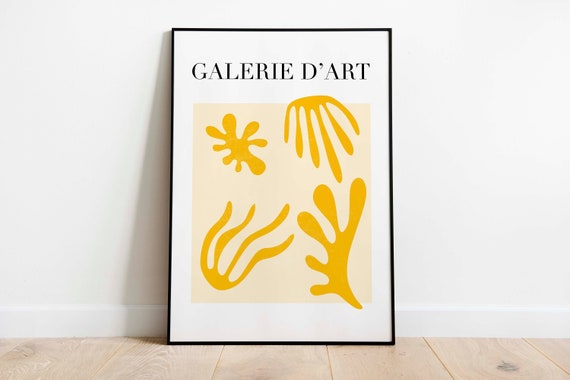The photograph captures a framed artwork resting on a light beige hardwood floor, leaning against a white wall. The frame is slender and black, approximately 10 by 18 inches in size. At the top of the white poster, there is thin black text reading "Galerie d'Art." Below this text, the central artwork features a light yellow background adorned with four abstract, orange shapes that resemble amoebas or corals. These shapes vary in design and size; the top left one is splat-shaped, the top right resembles a comb, the bottom left looks like a lute, and the bottom right is reminiscent of a frog's foot. The entire piece has a Picasso-esque, abstract quality, emphasizing unique and curious forms.